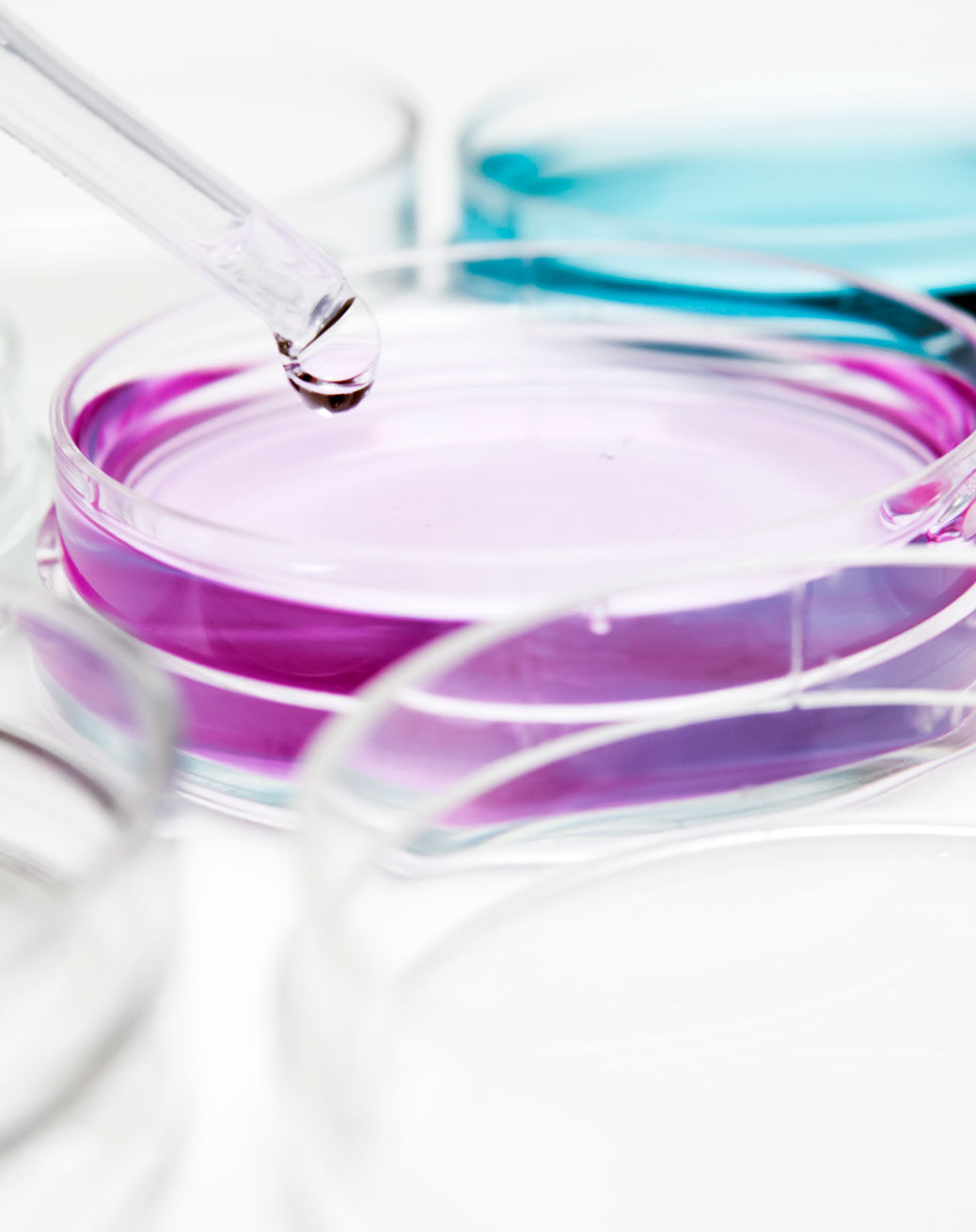In this detailed photograph, a liquid dropper is seen dispensing a single drop of clear liquid into a petri dish, hinting at a scientific experiment. The petri dishes are arrayed on a pristine white surface, showcasing varying colors and arrangements. Central to the image is a petri dish with a distinctive purple halo along its edges. Adjacent to it, in the upper right, is another petri dish, marked by a striking teal color. Two additional petri dishes occupy the lower left and lower right corners of the image, contributing to the symmetrical layout. The dropper extends from the upper left of the frame, emphasizing the meticulous process of adding a droplet into the central dish, which might contain clear liquid. The composition and elements suggest a scientific setting, although no individuals are visible, enhancing the focus on the experimental procedure itself.